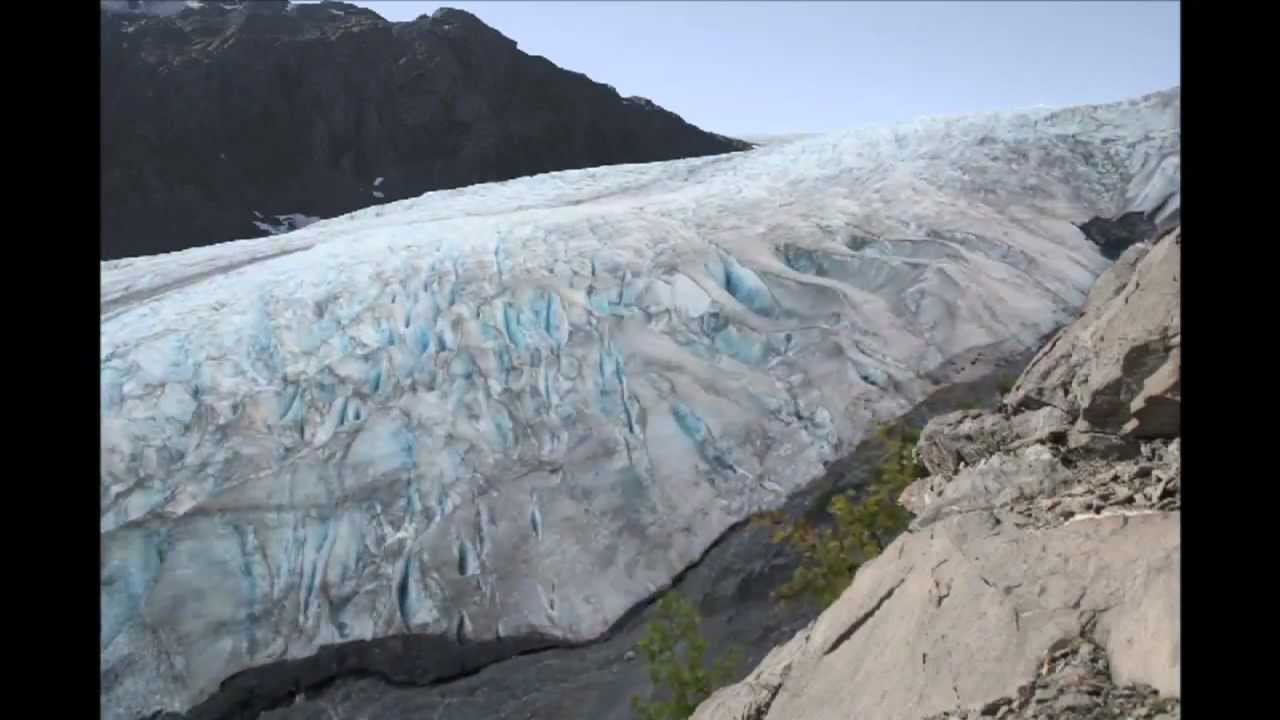The image depicts a mountainous landscape dominated by snowy and rocky features. On the left side, a snow-covered mountain is visible, possibly an ice glacier, with white and gray hues hinting at the possibility of ice. The center of the image is characterized by an austere, gray rocky terrain interspersed with patches of green moss, and a river runs at the base of the mountains, snaking through the rocky landscape. On the right side, a solid stone cliff devoid of snow rises prominently. In the top left corner, another smaller mountain with a snow-capped peak can be seen, indicating a cold environment. The sky above is a clear blue, suggesting daytime, and the overall scene appears starkly barren yet striking in its natural ruggedness. A black border frames the left and right sides of the picture. There are no people present in this desolate, rural location.